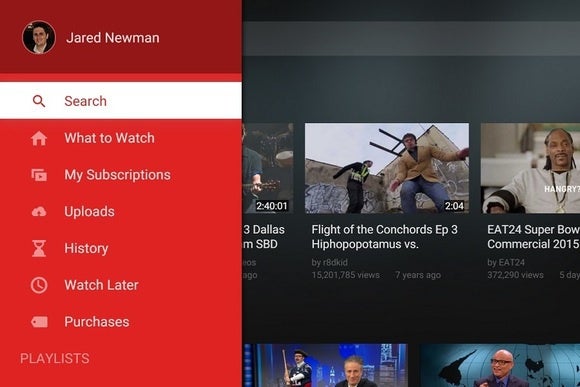Screenshot of a video hosting site profile belonging to subscriber Jared Newman. The left side features a long vertical section with Jared Newman's profile picture at the top, beneath which lie a search bar and several navigational options including: "What to Watch," "My Subscriptions," "Uploads," "History," "Watch Later," "Purchases," and "Playlists." This panel partially overlays the right side of the screen, which has a black background showcasing video thumbnails arranged in two lines.

Visible on the right side are selected thumbnails, although some are partially covered by the options menu. The first thumbnail is for "Flight of the Conchords, Episode 3: Hip Hopopotamus vs. Rhymenoceros," a 2-minute and 4-second video featuring an image of the two comedy duo members. This video was posted by user "RBD Kid." To the right of this, there's another thumbnail featuring a Super Bowl commercial from 2015, starring Snoop Dogg.